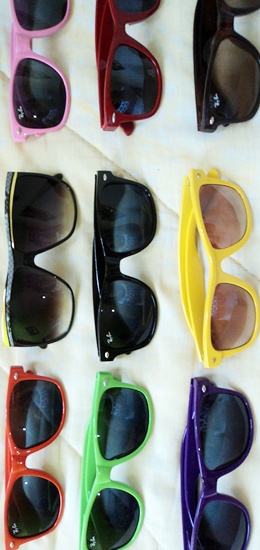The photograph displays a neatly arranged collection of nine pairs of sunglasses, laid out in a 3x3 grid on a white or vanilla-colored surface, which could be a table or quilt. The sunglasses are oriented horizontally with the arms facing to the left and lenses to the right. Starting from the top row, from left to right, the first pair of sunglasses has pink frames, followed by maroon-colored frames, and then black frames. In the second row, the leftmost pair has green frames with a yellow streak, followed by another pair with black frames, and then one with yellow frames featuring rose-colored lenses. The third and bottom row starts with red frames on the left, lime green frames in the middle, and purple frames on the right. All sunglasses appear to be inexpensive fashion accessories, differing mostly by frame color.